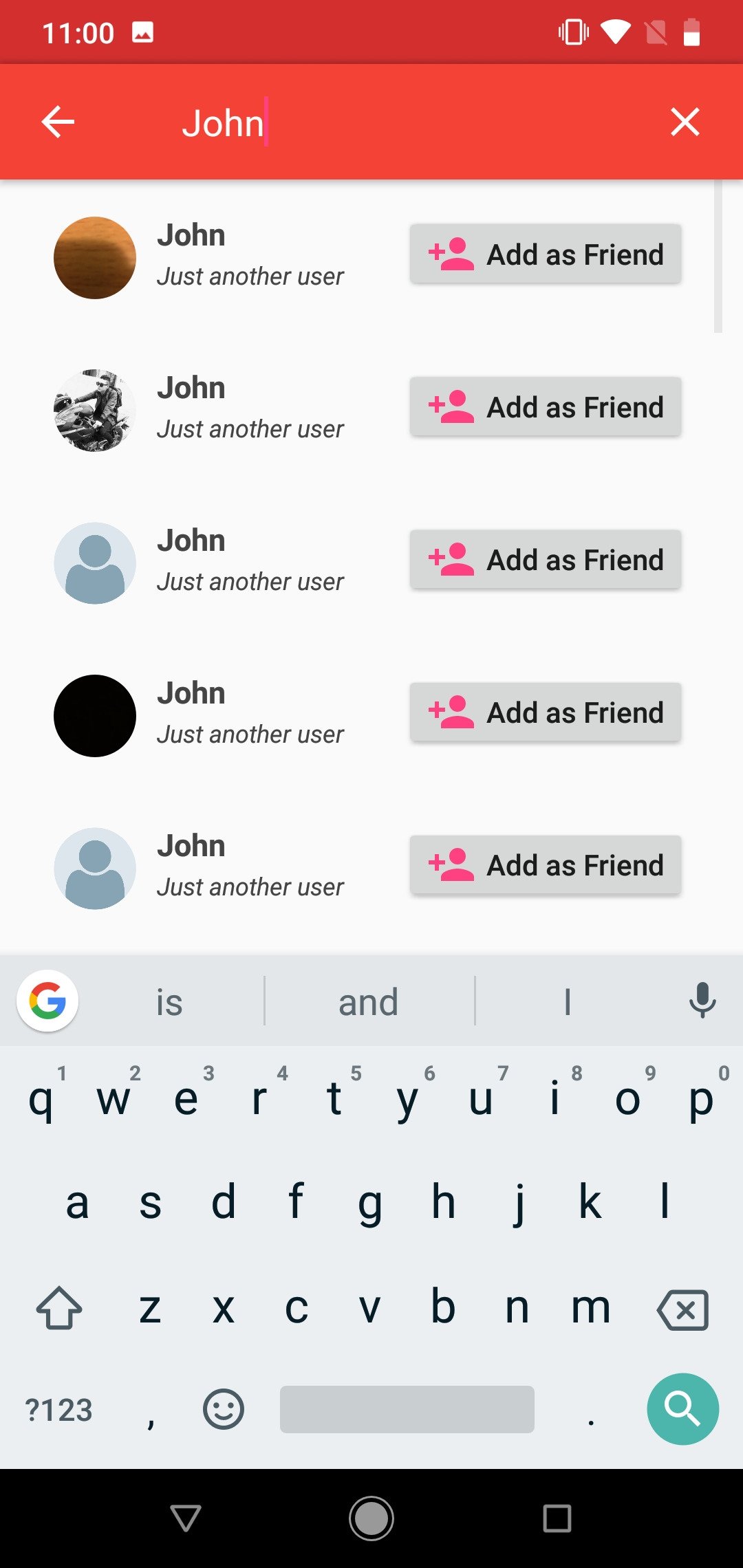A screenshot taken from a mobile phone displays a contact page for a user named "John." The header section includes a label 'John' at the upper top, with a left-pointing arrow for navigating back and an 'X' on the right, indicating the option to close the page. Below 'John,' the subtitle "just another user" is visible.

The list below the header features multiple entries, each labeled with 'John' and the same subtitle, "just another user." The first entry showcases a profile picture with an orange hue. The second entry is distinguished by a real person's photograph. Following that, there's a profile picture in black, succeeded by two generic icons depicting a circle with shoulders at the top.

Each entry has an adjacent feature—a pink icon of a person accompanied by a plus sign, alongside the label "add as friend." This pattern repeats consistently down the list. At the very bottom of the screen, a keypad is present for typing letters and numbers, indicating interactive input options.